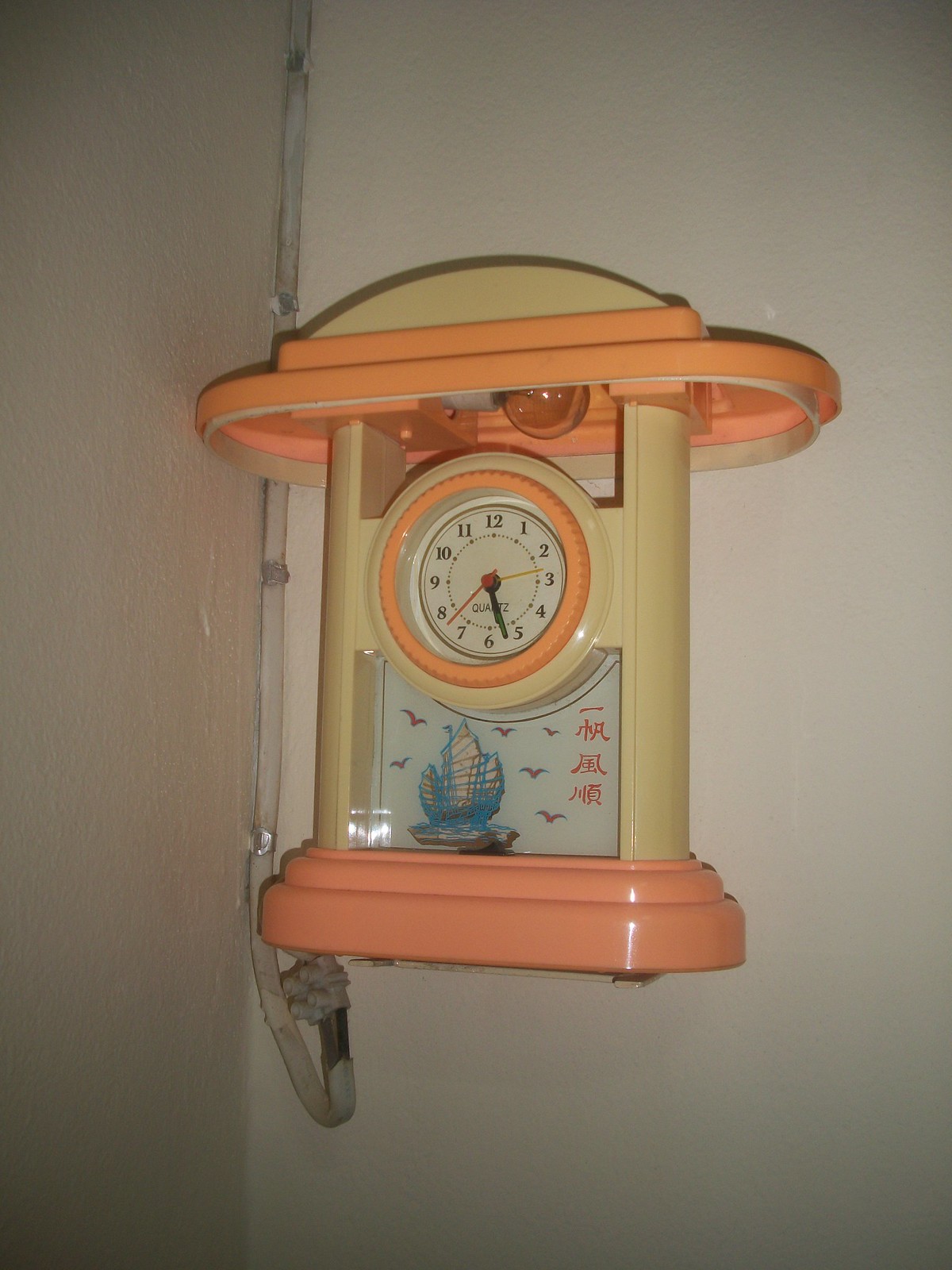This image features a close-up view of a vintage-style miniature clock encased within a decorative frame. The bottom portion of the frame is a unique blend of salmon pink and orange hues. Positioned above this colorful base is a vertically oriented, square-like structure with tan-colored edges. Below the clock face, there's an intricate design depicting a sailboat with brown hull, blue and white sails, accompanied by three red symbols to the right and a few doves flying nearby. The clock itself is framed by an orange ring. The numerals on the clock face range from 12 at the top, around full circle, returning to 12. The clock hands are currently positioned between the 5 and 6. The top of the clock features an orange section transitioning to a tan peak. The background wall to the left and behind the clock is painted a muted gray, providing a neutral backdrop that highlights the colorful and detailed clock.